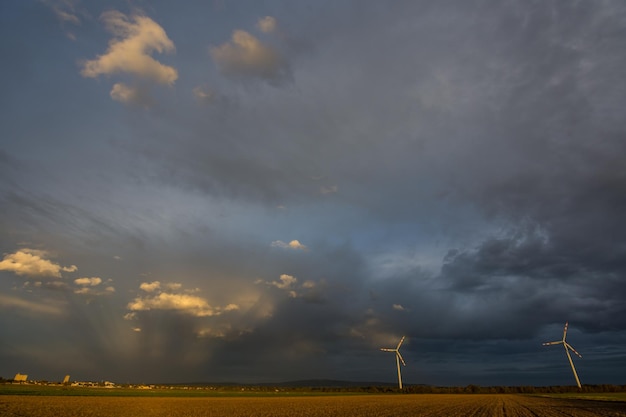In this outdoor scene, a vast golden field stretches across the forefront, possibly containing a crop, while adjacent greenery hints at another type of cultivation. Two towering modern wind turbines with three blades, designed to harvest wind energy, dominate the bottom right, standing tall against the expansive sky. The sky itself is a mix of turbulent weather, with dark, heavy clouds predominating, though patches of blue peek through occasionally. This menacing cloud cover suggests the imminent approach of a thunderstorm. Tiny, indistinct buildings or homes dot the far left, suggesting either a distant farm or the outskirts of a town. The overall atmosphere is bleak and ominous, casting a shadow over the entire landscape.